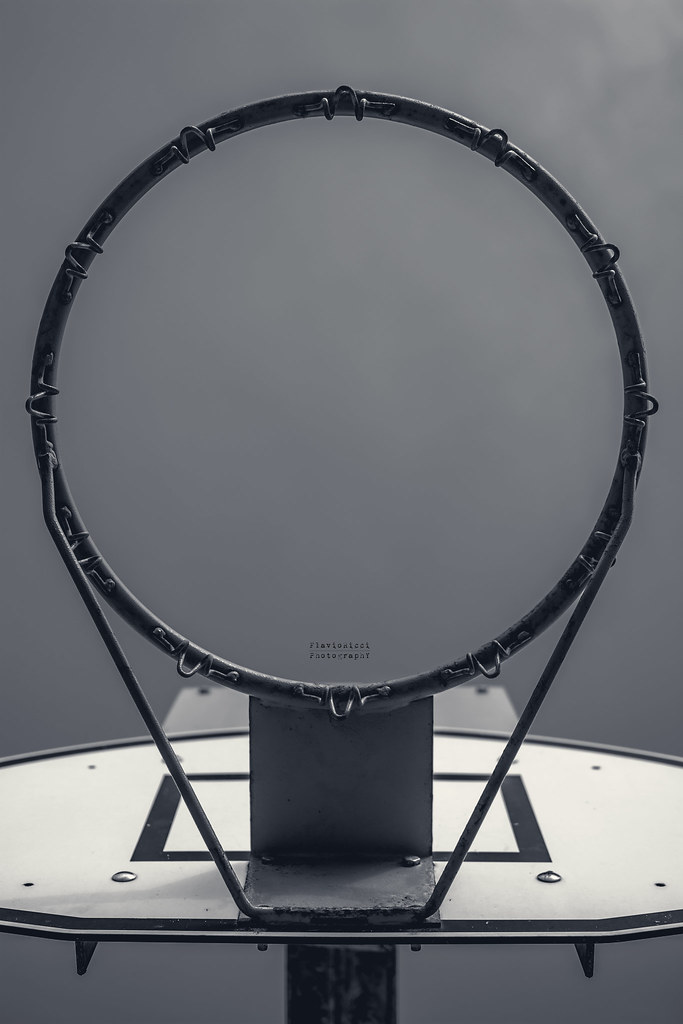The image is a black and white photograph taken from directly underneath a basketball hoop, looking up at the sky. The hoop is black without a net, and its hooks for hanging a net are visible. The backboard is the usual white with a black square in the center. The backdrop consists of dark gray clouds, giving the impression of an overcast day. Additionally, there's a faint text signature, "Flavio Ricci, photographer," on the bottom of the hoop, indicating the creator of the image. The overall composition suggests a stark, almost artistic quality, as if the scene might have been captured in a studio setting or with professional lighting.